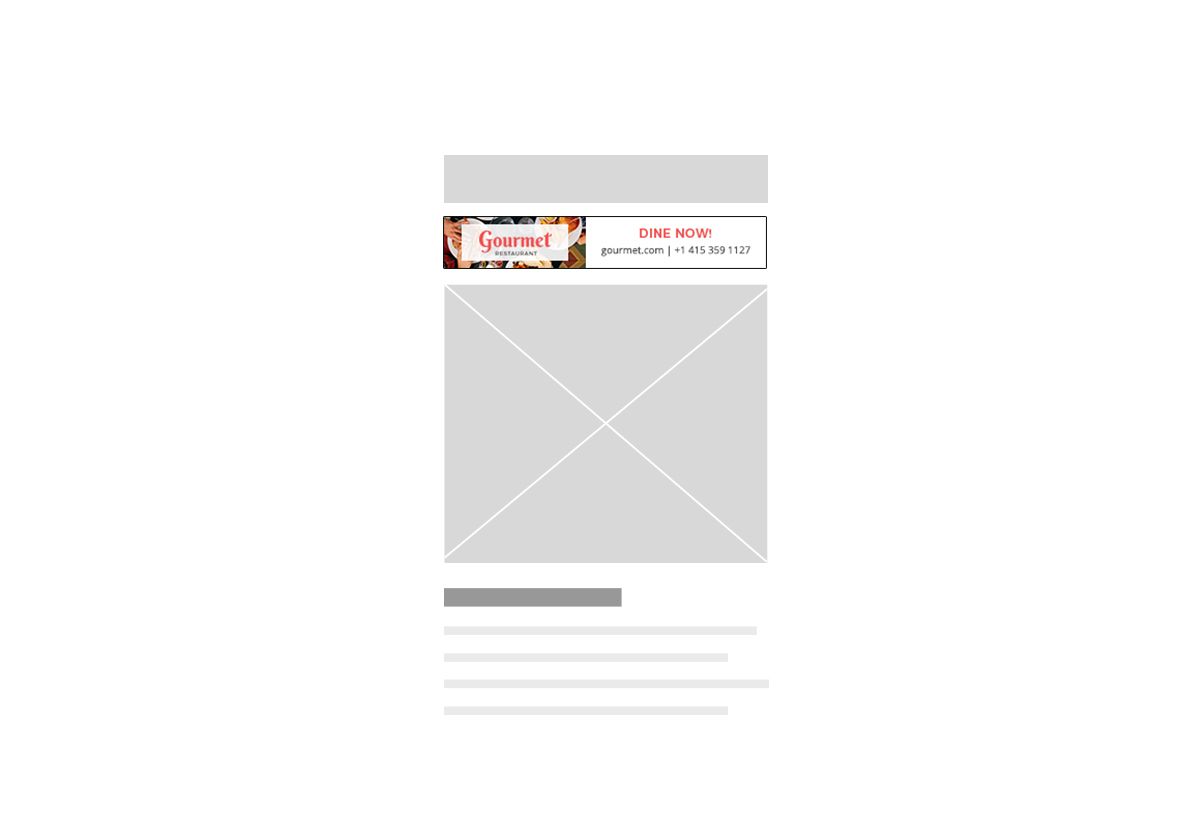The image appears to be a screenshot of a website currently under construction or with information intentionally redacted, presenting a minimalistic and unfinished appearance. At the top of the page, there is a wide, medium-toned gray area bordered by a thin black line, serving as a placeholder for a banner. This banner, which contains some information, is divided into two sections.

On the left third of the banner, there is an image showing a top-down view of food on a table, partially covered by a white rectangle. Within this rectangle, the word "GOURMET" is prominently displayed in red letters, with "RESTAURANT" written below in black text. To the right of this image, the text "DINE NOW!" is boldly written in red, followed by the information "gourmet.com" and a contact number "+1 415-359-1127" written in black beneath it.

Descending further down the page, a gray square is visible, distinguished by two intersecting white diagonal lines forming an 'X' pattern. Below this gray square, a dark gray bar spans from the left edge of the page to the center, covering half of the page's width. Within this dark gray bar, there are five lighter gray lines arranged to resemble paragraphs, though these lines are purely decorative and do not contain any actual text.